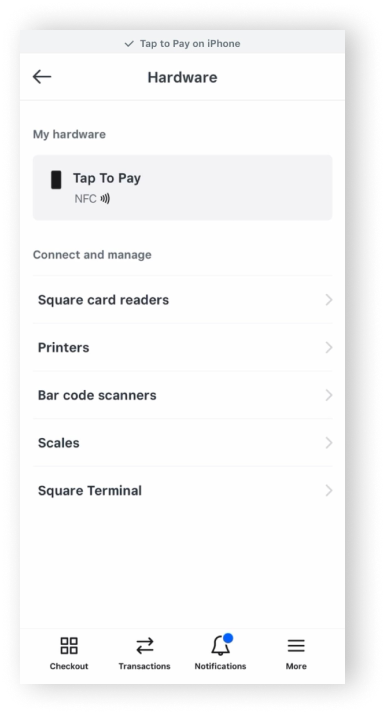The image showcases a detailed interface of a point-of-sale (POS) application, likely from Square or a similar service. The central theme of the interface is the "Hardware" management page, emphasizing the system's capability to support various devices and accessories. Key features include the option to set up "Tap to Pay," highlighting Near-Field Communication (NFC) technology for contactless payments. 

The interface offers several options:
- **Square Card Readers:** Options for connecting and managing card readers to facilitate transactions.
- **Printers:** Settings for connecting and managing printing devices, crucial for receipts and order tickets.
- **Barcode Scanners:** Compatibility settings to connect barcode scanners for streamlined product scanning.
- **Scales:** Options for integrating scales, primarily useful for businesses that sell products by weight.
- **Square Terminal:** Management options for Square Terminal devices, enabling comprehensive POS functionalities.

The navigation menu at the bottom consists of several tabs:
- **Checkout:** Likely redirects users to the main checkout page to process transactions.
- **Transaction History:** Provides a detailed record of past transactions for reference and bookkeeping.
- **Notifications:** Enables access to alerts and updates, possibly related to software, payments, or hardware connectivity.
- **More:** Presumably a section for additional settings, help resources, or advanced features.

Overall, the image reflects an intuitive and organized hardware configuration page designed to support various POS components, facilitating a seamless transaction process through NFC-enabled tap payments on an iPhone.